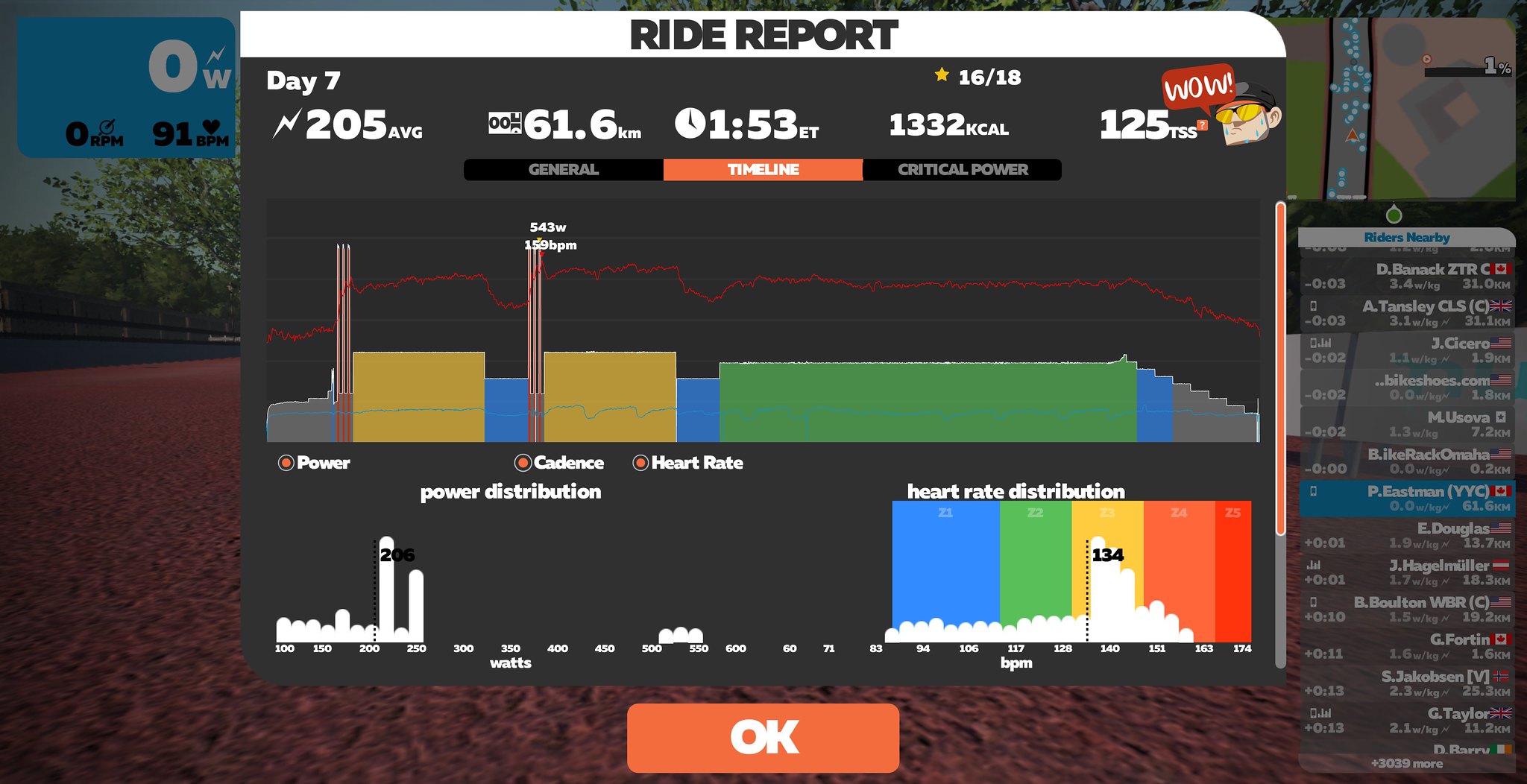The image is a detailed screenshot from a high-tech biking app or website, featuring a "Ride Report" for Day 7, possibly from a gamified indoor exercise bike system like Peloton. The main section highlights key metrics: an average of 205 units (likely power in watts), 61.6 kilometers covered, a time of 1:53 ET, and 1,332 calories burned. Additional data includes a Training Stress Score (TSS) of 1.25. Graphical elements include a line graph and bar graphs in various colors (yellow, green, and blue) showing detailed statistics for Power, Cadence, Heart Rate, and Power Distribution. To the right, there is a list of participants, marked with different flags, indicating competition standings at the end of Day 7. The interface is visually rich, with an orange "OK" button at the bottom center. A small map is also visible in the background, adding to the gamified experience.